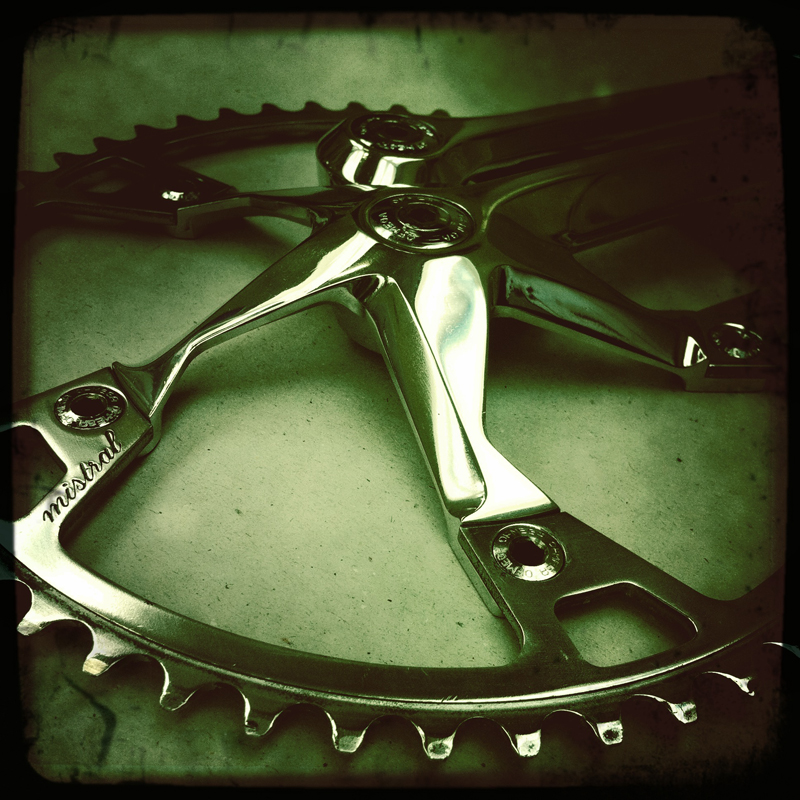The image depicts a large and hefty, high-polished silver metal gear resting on a concrete floor with a greenish tint. The gear, which has five joints and little metal teeth along its circular edge, is partly shadowed, making it appear darker, almost black, towards the front right. Engraved on it are the words "Miss Trat." A metal wrench can be seen lying on top of the gear. The lighting in the photograph shines predominantly on the middle of the gear, casting shadows and adding to the intricate texture and detail. The scene appears to be indoors, possibly in a garage, with limited lighting contributing to a dim, yet clear, setting. The silvery metallic gear and cement floor contrast sharply, highlighting the gear's robust, industrial design.